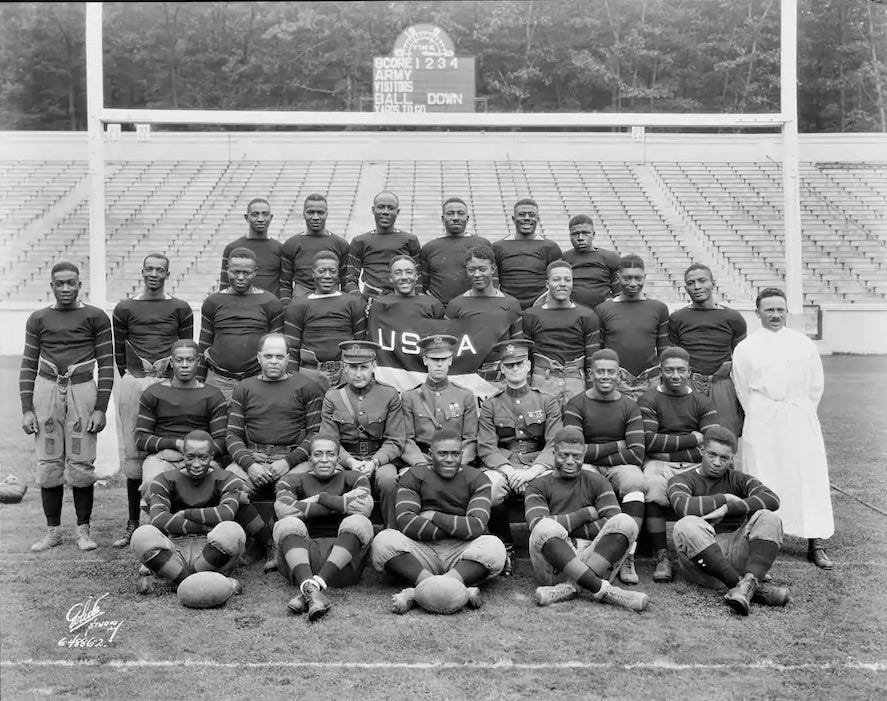This black-and-white photograph, likely from the early 20th century, captures an historic moment for an all African-American football team. The image, possibly from the 1920s or 1930s, shows approximately 15 to 16 players and is set in front of a goalpost, with empty bleachers visible in the background. Three men in military uniforms sit prominently in the middle of the team, suggesting a military academy affiliation. To the side stands a figure in a white coat or robe, possibly indicating a coach, doctor, or religious official. The scoreboard behind reads "Army vs. Visitors," and a small sign or flag displaying "USA" can also be seen. There is an indistinct drawing or signature in the lower left corner of the photograph.